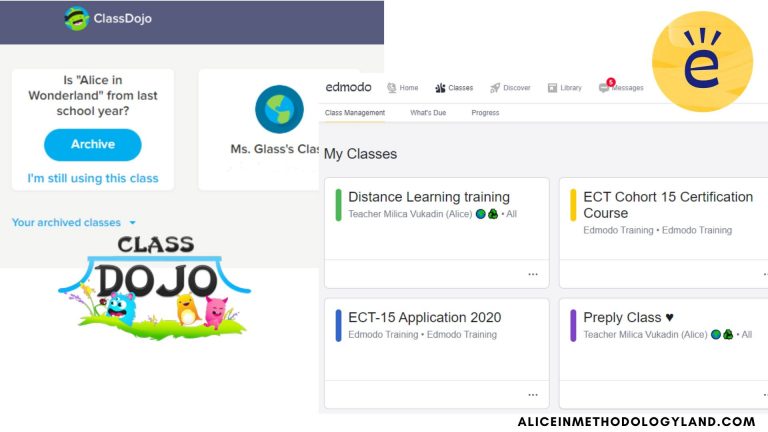The image is a colorful landscape screenshot of a web page layout for ClassDojo, an educational platform. Dominating the screen is the distinct ClassDojo logo, characterized by a calligraphy-style font with clear Asian influences, possibly Japanese or Korean. The logo is written in bold, dark black, all capital letters, exuding a traditional aesthetic. Nestled between the words "Class" and "Dojo," there is a striking blue line that curves like the roof of a traditional Japanese house, flat on top with elegantly curved sides.

Beneath this roof-like design are whimsical, anime-inspired characters reminiscent of Hello Kitty creatures. These adorable, smiling monsters appear joyous and animated, suggesting an engaging and fun learning environment. They dance gleefully in a lush green space, adding a touch of vibrancy and happiness to the visual.

The web page is filled with various interactive elements and navigation options. Users can browse through different sections such as an "Alice in Wonderland" archive from the previous school year, or access a list of classes. Other options on the page include selecting distance learning training, among other educational tools and resources. The overall design and content of the page evoke a sense of cheerful productivity and user-friendly navigation.